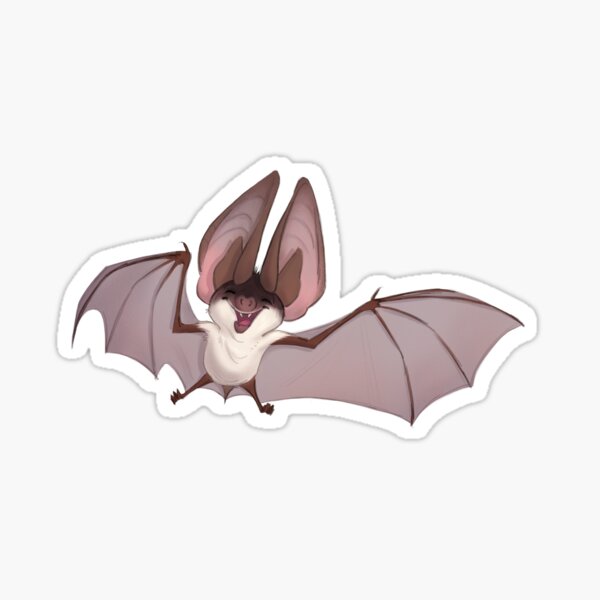The image features a cartoonish depiction of a bat against a white background, resembling a cut-out decal or sticker. The bat, centrally positioned and slightly rotated clockwise by about 15 degrees, is outlined in white and showcases exaggerated, kidney-shaped ears that are nearly as long as its body. These ears have dark gray outer edges and an inner part matching their elongated shape. The bat's body is furry and cream-colored, with an expressive face sporting an open mouth that appears to be smiling, revealing its fangs and a hint of its tongue. Its outstretched wings, light gray with darker veins and edges, extend towards the left and right sides of the image, while its feet point downward. The bat’s face, with visible eyes, snout, and a black upper portion, along with its spread-out stance and detailed features, gives it a lively, almost caricature-like appearance.